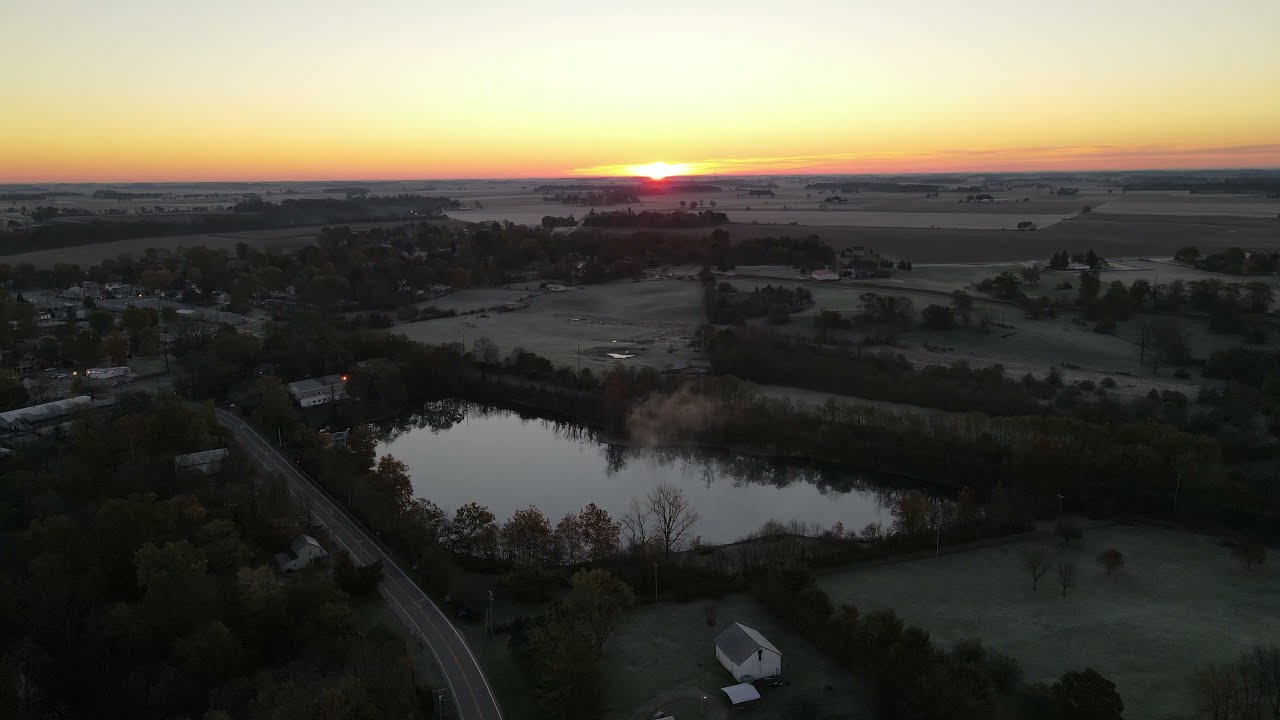An aerial photograph captures a serene rural landscape at either sunrise or sunset, with the sun positioned prominently on the horizon, casting a beautiful gradient from a bright yellow orb to an expansive orange hue along the horizon line, eventually fading to a soft gray-blue at the top of the image. The scene features a tranquil pond at the center, surrounded by a reflection of encircling trees. To the left, a two-lane road winds from the bottom left corner, curving up and to the left, bordered by groves of trees and clusters of buildings that likely represent a small commercial area. Adjacent to this road lies a grassy field divided by another line of trees, with a small, white farmhouse on one lot and a barren field on the other. In the distance to the right of the pond, rolling fields and scattered trees stretch towards the horizon. The entire landscape exudes a peaceful, countryside charm, accentuated by the soft, dim light of the early morning or late afternoon, highlighting the quiet beauty of rural life.